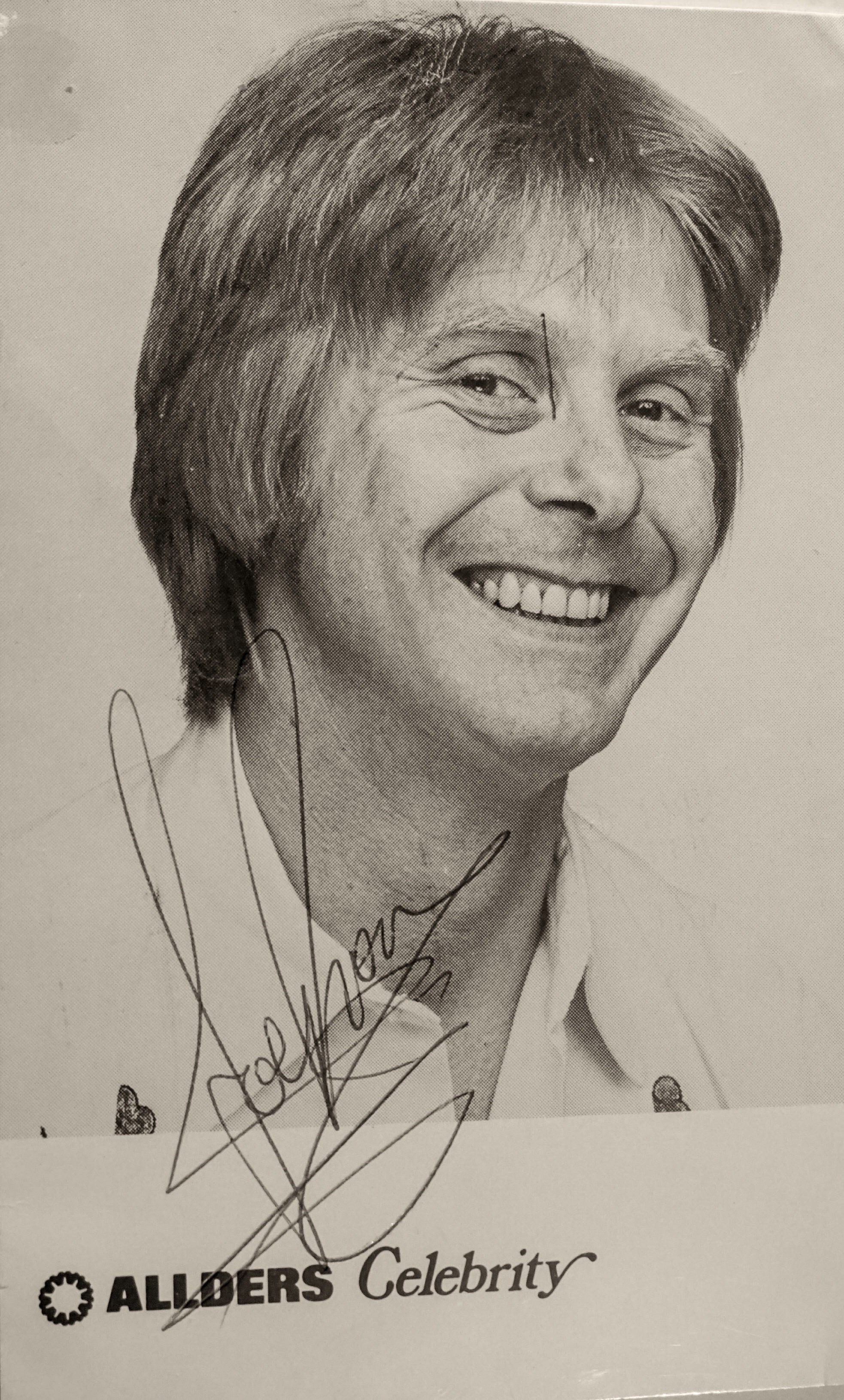The image displays a black-and-white photograph of an older, Caucasian male celebrity with mid-length, medium-colored hair draped down. His teeth are showing, and his nose is somewhat crooked. The man is wearing a white shirt that is unbuttoned at the top, revealing partial symbols on both the left and right sides, though these symbols are cut off and not fully visible. His dark eyes add to the intensity of the gaze. The photograph features a signature, possibly reading "Joe Brown" or something similar, autographed directly over the man's face with a pen. Below the photo, there is a white section with a circular bumpy logo resembling a sun inside, and next to it, in black capital letters, the word "Alders" followed by "Celebrity" in regular black text. The backdrop of the photograph is plain white.